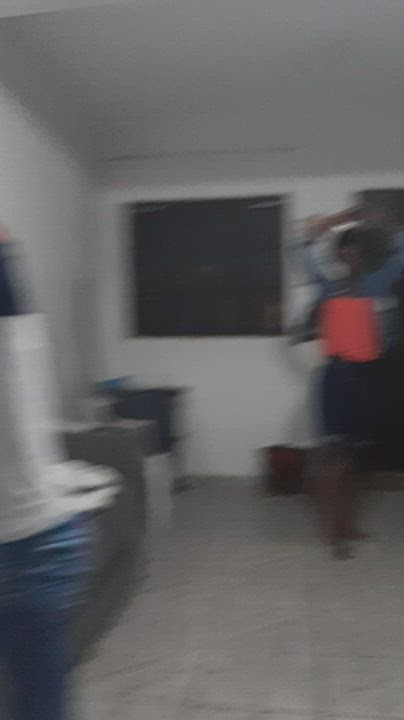The photograph, although quite blurry and out of focus, captures the interior of a room with a gray floor, white walls, and a white ceiling. Centered on the back wall is a notable black rectangle, which includes white stripes extending slightly towards the center from the top left and top right edges, suggesting it might be a window. To the right of this rectangle is a person with their arms raised above their head. They appear to be dressed in a red shirt, a blue coat, and blue shorts. On the left side of the image, near the gray floor, there is a black couch. Despite the low quality of the photograph, these distinctive elements can be discerned.